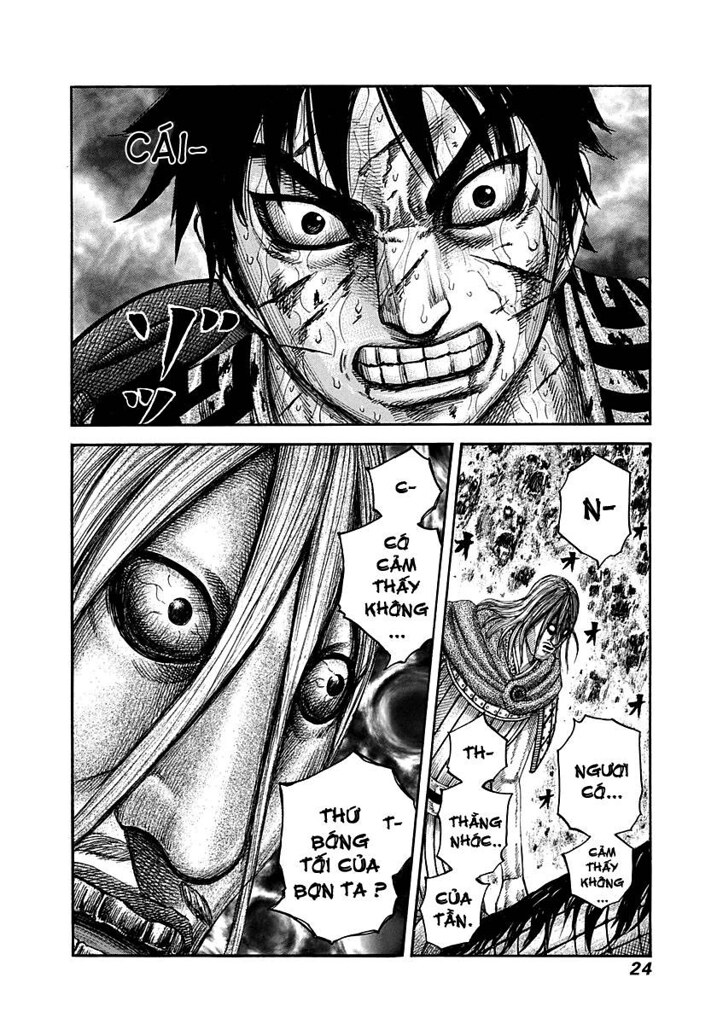This is a black-and-white page from a graphic novel, specifically page 24. The text appears to be in Vietnamese, enhancing its distinct anime-like feel. The top panel is a dramatic close-up of a distressed man with medium-length black hair, his eyes wide with fear, and his face glistening with sweat and possibly tears. His mouth is clenched, and his hair covers part of his eyes. Below, the page is divided into two side-by-side panels. The left panel features a terrifying figure with long, white hair and intensely wide-open, bloodshot eyes. His expression is almost lifeless, with prominent veins stretching out from the corners of his eyes and dark, menacing teeth visible. In the bottom right panel, this same man is seen from a distance, looking downwards. Behind him, the sky is filled with disturbing, ghostly demon faces emerging from the shadows, alongside debris and human bodies that add to the chaotic and eerie atmosphere. The detailed illustration captures a sense of horror and tension across all panels.